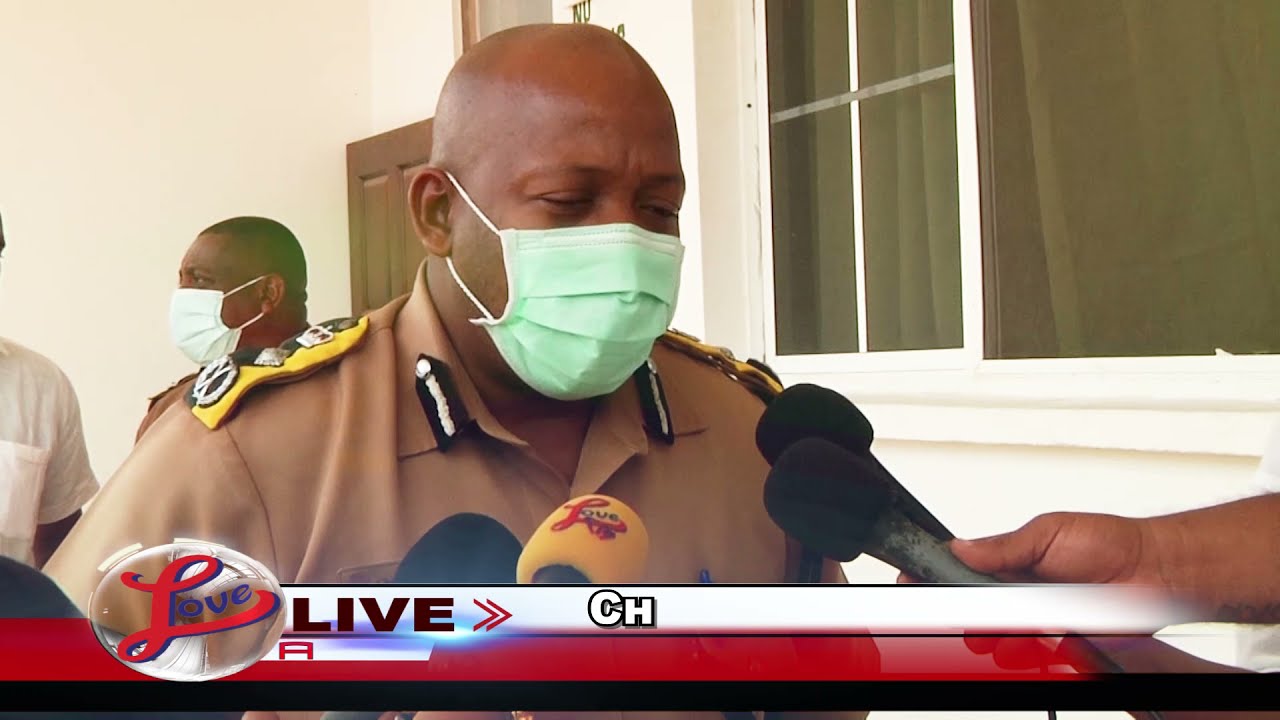This color photograph depicts a television news broadcast scene featuring an African American man in a military uniform, presumably an officer, wearing a green medical mask. He stands at the center, facing a bank of four microphones with yellow and black covers, indicative of an ongoing interview. The man has a bald head and is attired in a brown uniform adorned with yellow and green emblems on the shoulders, silver decorations, and black collar tabs with silver trim. 

Behind him, other elements of the environment are visible: a white-framed window with curtains and a brown wooden door set in white walls. To his right, another uniformed man, also masked, converses with an individual in a barely visible white short-sleeved shirt. The television graphic at the bottom includes red and blue lettering, a circle with the word "Love," and the words "Live" and "CH" displayed in white on a white band, above red and black bands. A human hand holding one of the microphones can be seen in the lower right corner.